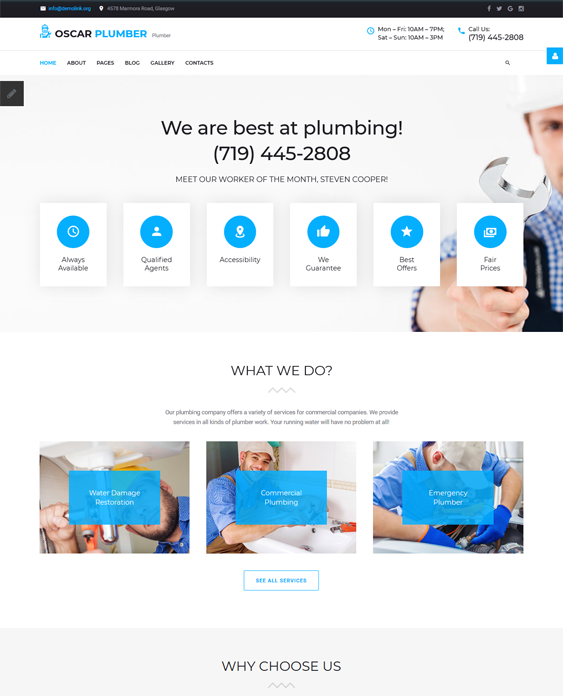The web page for the business "Oscar Plummer" features a streamlined design with a clean, all-white background. At the top of the page, the business name is prominently displayed, followed by the operational hours: Monday to Friday from 10:00 AM to 7:00 PM, and Saturday to Sunday from 10:00 AM to 3:00 PM. Below the hours, there's a contact phone number: 719-445-2808.

Further down, the navigation menu includes links to various sections: Home, About, Prices, Blog, Gallery, and Contacts. The main visual element is an image of a gentleman in a hard hat holding a wrench, accompanied by the text "We are best at plumbing" and the repeated phone number.

The page also highlights Stephen Cooper as the "Worker of the Month" with a mention next to his picture.

Additional features include several informative boxes with rounded icons, depicting services and guarantees such as "Always Available," "Qualified Agents," "Accessibility," "We Guarantee," "Best Offers," and "Fair Prices."

Following these, there's a section titled "What We Do," although the description is too small to read. It is accompanied by three images of a plumber at work, illustrating different plumbing tasks. The first box below these images lists services including "Water Damage Restoration," "Commercial Plumbing," and "Emergency Plumbing," with a prompt to "See All Services" and an additional section on "Why Choose Us."